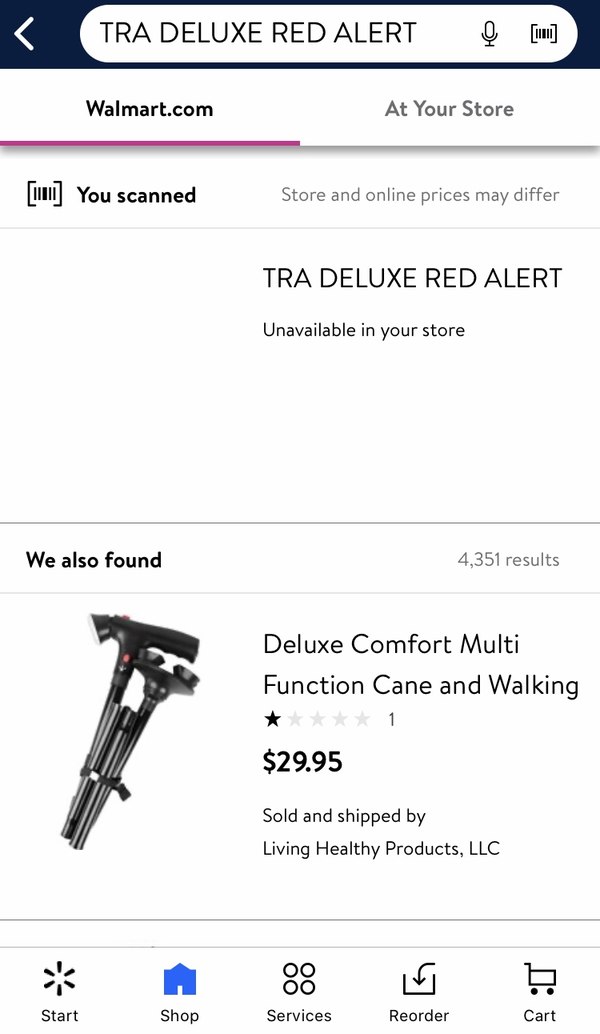The image displays a screenshot of the Walmart mobile app. At the top of the screen is a search bar containing the query "TRA Deluxe Red Alert." The app indicates that the "TRA Deluxe Red Alert" product is unavailable at the user's selected store. Instead, the app suggests an alternative item listed as "Deluxe Comfort Multifunction Cane and Walking Stick," priced at $29.95. Notably, this alternative product has received a single review, rating it one star. The item is sold and shipped by Living Health Productions LLC. At the bottom of the app interface are five navigation buttons: Home, Shop, Services, Reorder, and Cart, providing standard app functionality. Overall, the screenshot reflects a typical product search experience within the Walmart mobile app, specifically for a walking cane.